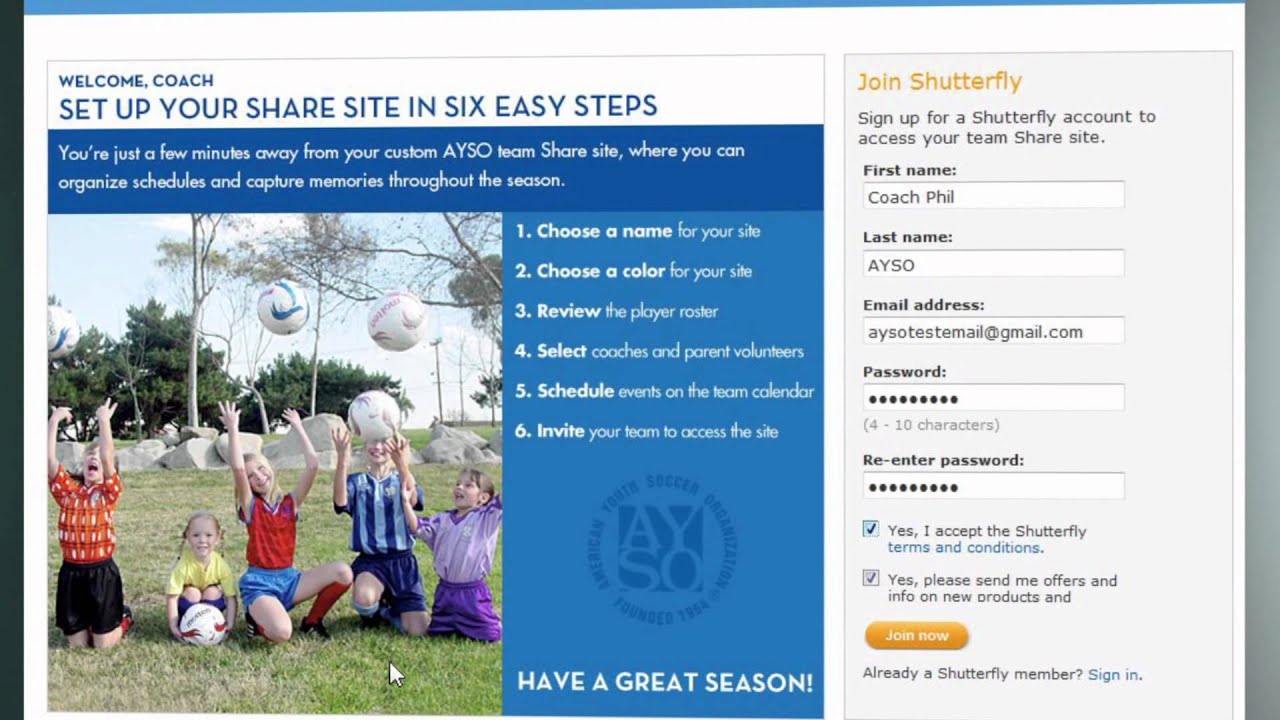Screenshot Description: Shutterfly Website Builder for Soccer Coaches

This screenshot captures the interface of Shutterfly's website builder tailored for soccer coaches. The layout is divided into two primary sections.

**Left Section: Share Site Setup Steps**
- **Header:** "Welcome Coach! Set up your Share Site in Six Easy Steps."
- **Steps List:**
  1. Choose a name for your site
  2. Choose a color for your site
  3. Review the player roster
  4. Select coaches and parent volunteers
  5. Schedule events on the team calendar
  6. Invite your team to access the site
- **Footer Message:** "Have a great season!"
- **Visuals:** Below the header is an engaging image of five young girls joyfully throwing soccer balls into the air. Each girl sports a unique uniform: 
  - Blue striped shirt
  - Purple shirt
  - Red shirt
  - Orange-red shirt with a white design
  - Yellow shirt

**Right Section: Join Shutterfly Form**
- **Prompt:** "Join Shutterfly"
- **Instructions:** "Sign up for a Shutterfly account to access your team Share Site."
- **Form Fields:**
  - First Name: [Coach Phil]
  - Last Name: [AYSO]
  - Email Address: [AYSOTestEmail@gmail.com]
  - Password: [••••••••]
  - Re-enter Password: [••••••••]
  - Two acceptance checkboxes
  - Orange "Join Now" button

This detailed walkthrough is designed to help soccer coaches efficiently set up their team’s share site and foster a cohesive team environment.